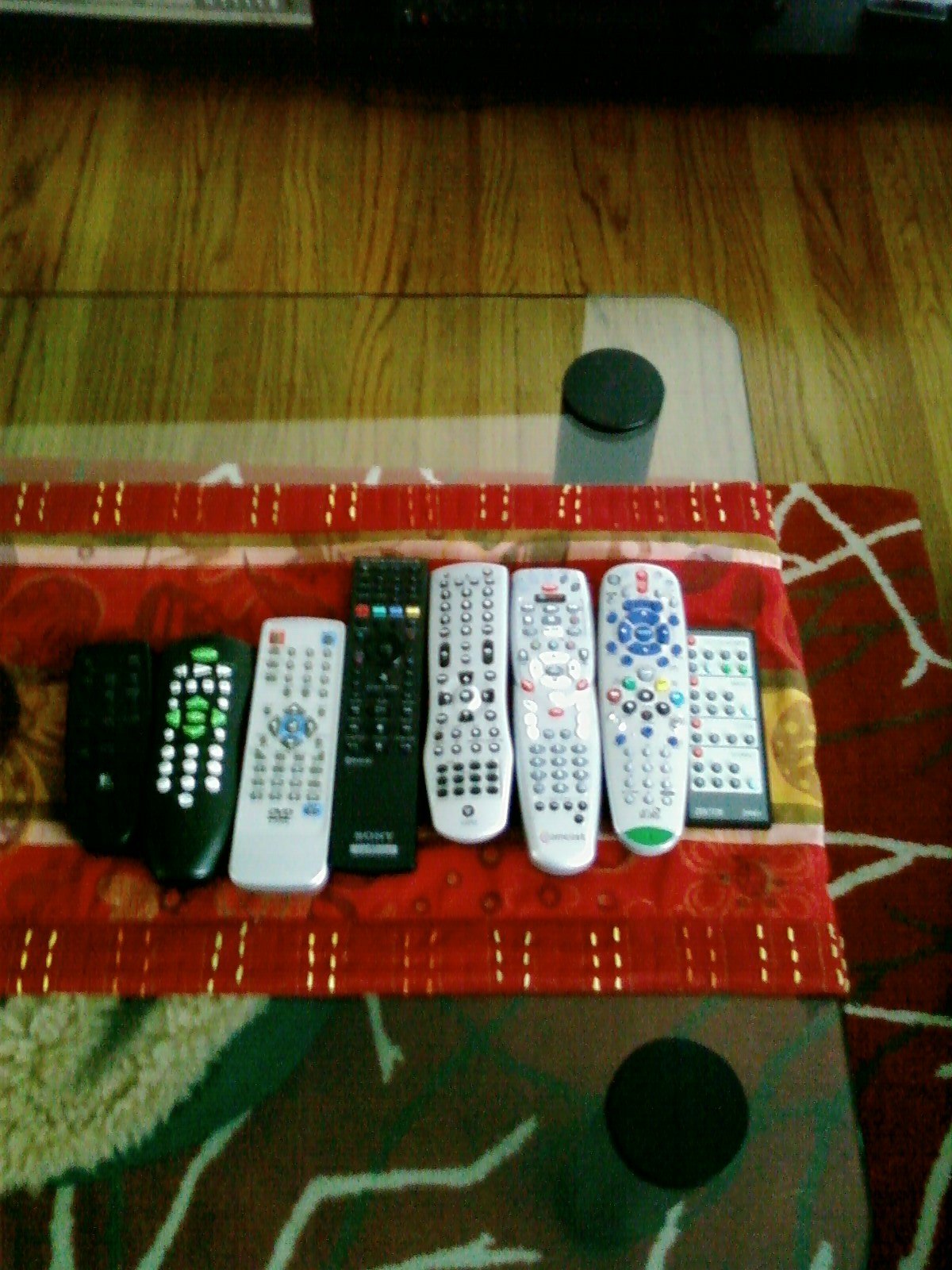The image is a detailed photograph taken in portrait orientation, capturing a top-down view at a slight 45-degree angle. The focal point is a row of eight remote controls laid out horizontally on a piece of red fabric which rests on a glass coffee table. These remote controls, used for various devices such as televisions, satellite TV boxes, and hi-fi systems, vary in size, shape, and style. Some are thicker and some are flatter; they feature a mix of colors with black, silver, and grey fronts, and multicolored, grey, or black buttons.

The glass coffee table, clear with round black discs at the corners where the legs attach, reveals an intricate setup beneath it. There is a plush circular dog bed partially obscured by the red cloth, and the table rests on a dark red rug with white twig-like patterns interspersed with brown.

In the top portion of the image, the wooden flooring, consisting of mid-brown tan planks, frames the scene, creating a warm and inviting living room setting. The meticulous arrangement and the blend of textures and colors provide an orderly yet homely ambiance.